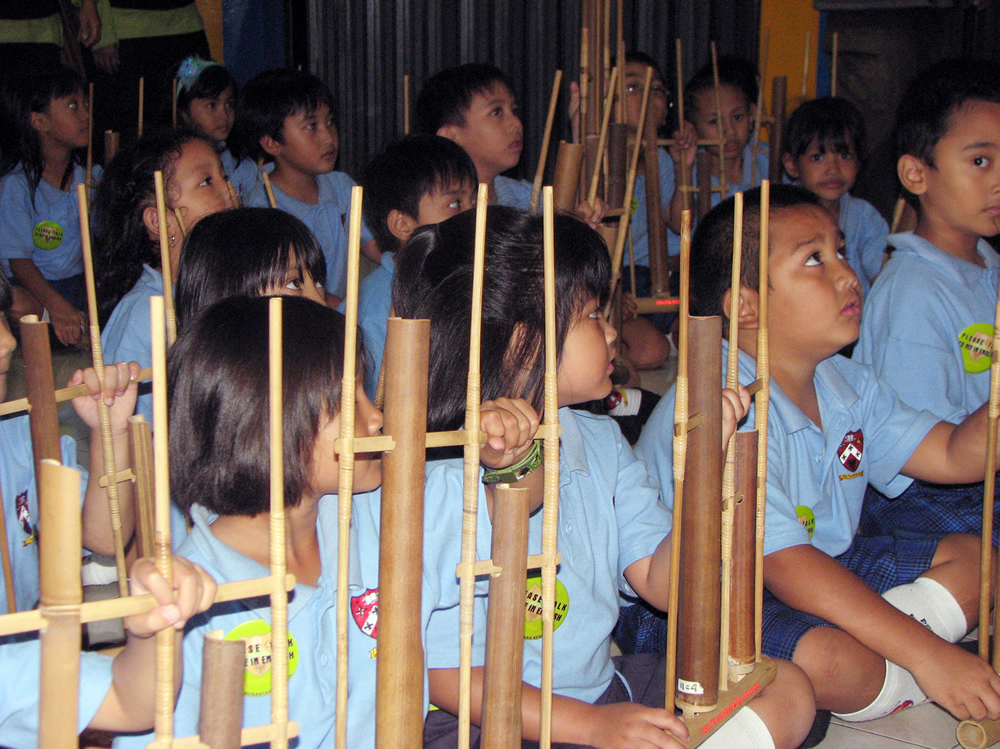This color photograph captures a group of school children, likely of Asian descent, sitting cross-legged on the floor in a dimly lit classroom in the Philippines. The children, dressed in a uniform consisting of light blue short-sleeved collared shirts with a red and blue plaid crest on the right chest and a green circular patch on the left, each wear blue plaid bottoms—shorts for the boys and either skirts or shorts for the girls—paired with white socks. Each child holds a wooden apparatus constructed from three wooden rods and two brown cardboard tubes anchored on a wooden base, suggesting a science project or craft activity. The children, arranged in approximately four orderly rows, are focused intently on something off-camera to the upper right, likely their teacher, except for one child on the far right who gazes directly at the camera, creating a sense of connection. The mixture of ambient light highlights the front rows more prominently than the back, adding depth to the image.